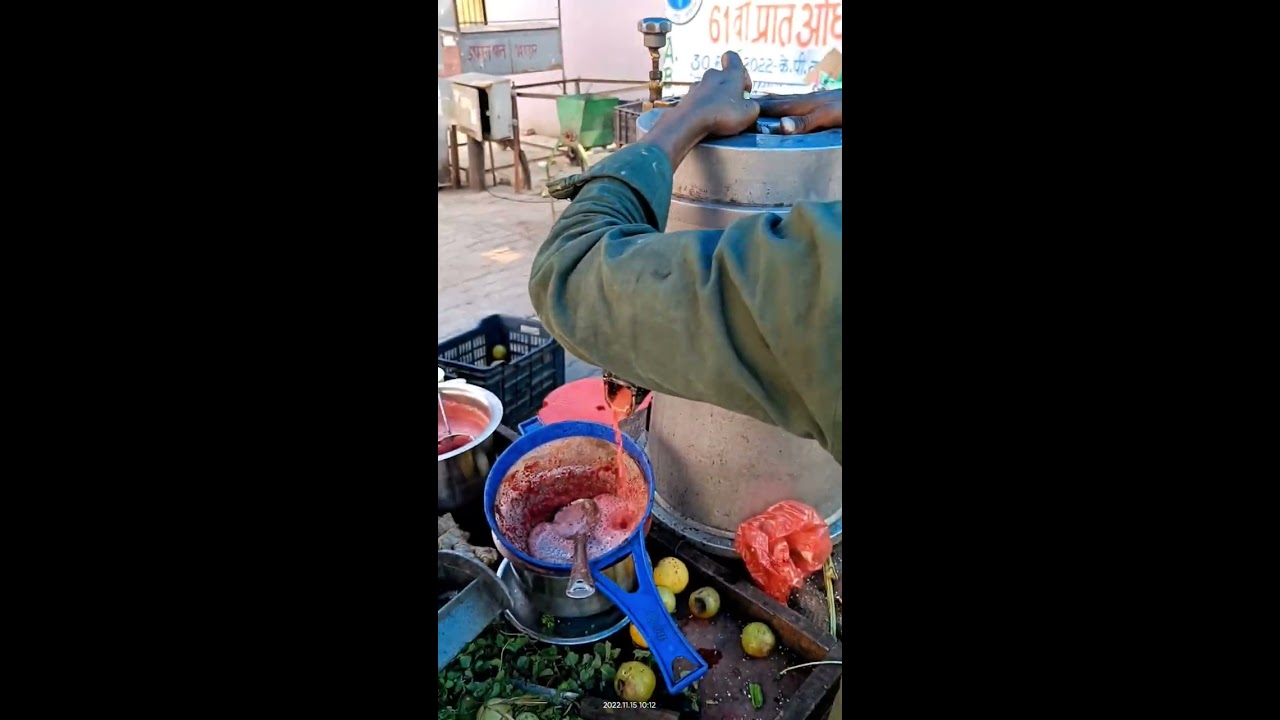This rectangular image is divided into three sections vertically, with the left and right thirds being solid black, framing a central photograph. The central photograph portrays an outdoor scene, seemingly in a primitive village. A dark-skinned street vendor, wearing an army green long-sleeved jacket, is partially visible, primarily by his left arm as he interacts with a tall, silver stock pot with a lid.

Around the vendor, there is a cooking area with various food items. In the bottom left, different types of food are visible, including light gray crab apples and watercress. A prominent blue pot containing a pinkish substance with a spoon in it suggests he is preparing food. Other smaller pots with similar pink contents surround the area. 

The background features a rough cobblestone road, a shopping cart, and the side of a gray concrete building adorned with text and images, possibly in a foreign language. The scene suggests an early morning preparatory activity at an outdoor food stand, awaiting the day's business.